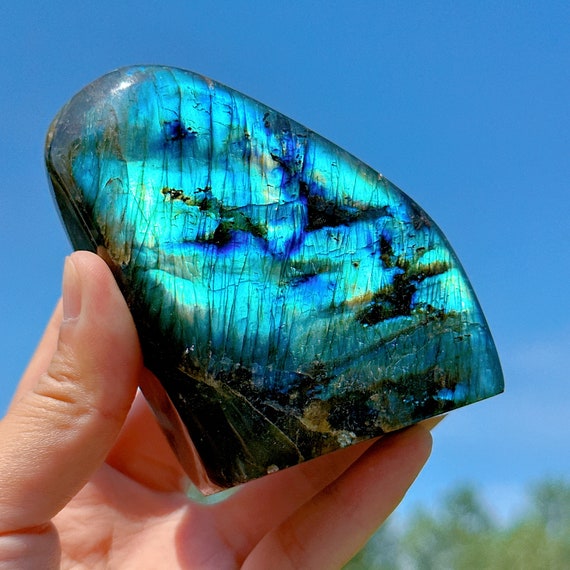In this photograph taken outdoors on a bright, clear day with a blue sky and a blurred line of trees in the background, the main focus is an individual's left hand holding a remarkable rock. The rock exhibits an intriguing blend of aqua, dark blue, green, and black colors and has an exceptionally shiny, almost holographic appearance. Likely polished, its bottom is flat and straight, suggesting it could be manufactured or artificially cut, while the top and right edges are naturally rounded. There's a subtle hint of gold within some cracks, giving the sense that different hues could emerge if rotated in the sunlight, enhancing its prism-like allure.